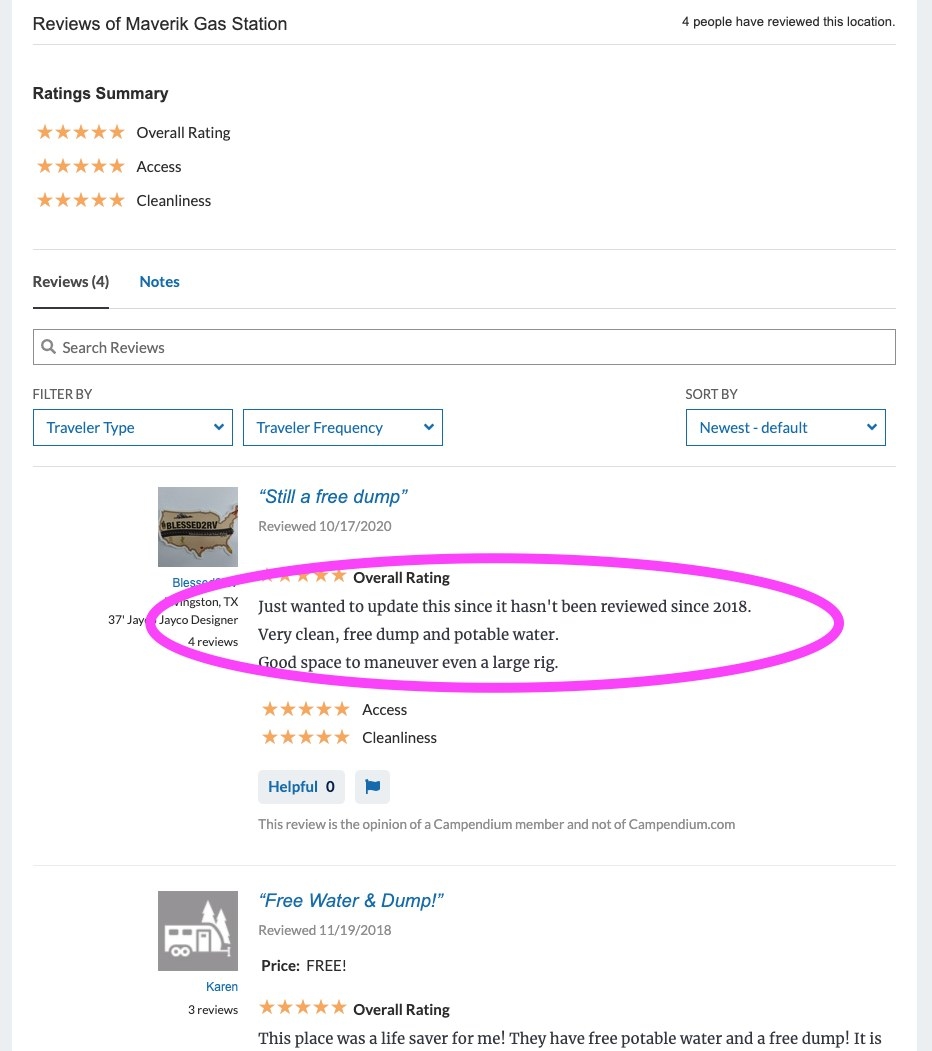The image displays a detailed review page for Maverik Gas Station, showcasing its highly-rated amenities. The top of the page is marked with the title "Reviews of Maverik Gas Station," indicating that four people have reviewed this location. The ratings are neatly separated by categories: an overall rating of five stars, five stars for access, and five stars for cleanliness.

A variety of filters can be applied to the reviews, such as travel type, travel frequency, and newest reviews first. The latest review, dated October 17, 2020, highlights the station's excellent facilities with an overall rating of five stars. The reviewer commends the station for its cleanliness and ample space for maneuvering large rigs, stating, "Just wanted to update since it hasn't been reviewed since 2018. Very clean, free dump, and potable water. Good space to maneuver even a large rig." Both access and cleanliness received five stars.

Another review from November 19, 2018, by a user named Karen, also gives the location a five-star rating. She praises the station as a "lifesaver," noting the availability of free potable water and a free dump station. Her review reinforces the idea that this gas station is particularly suitable for campers and RV travelers needing to dump waste and refill water supplies.